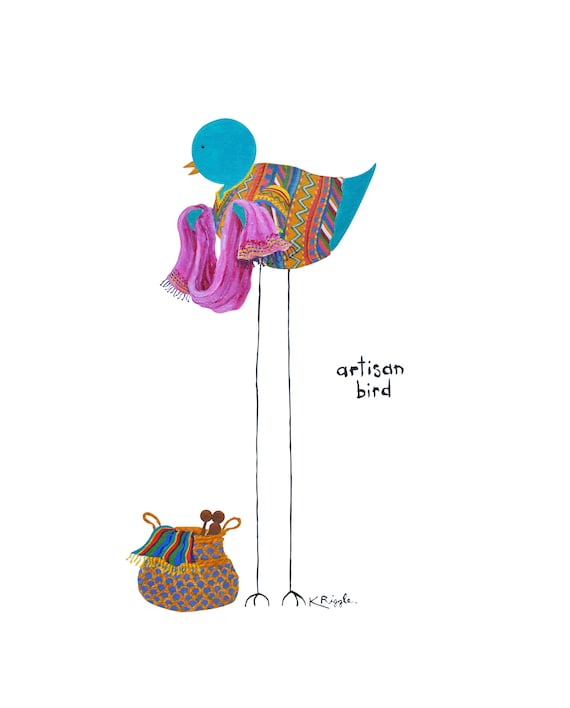In the image is an illustration of an "artisan bird," as indicated by the text in lowercase to the left of the image. The background is entirely white, setting a clean stage for the artwork. The bird, located at the top of the image, is a blue bird with a circular head featuring a very tiny black eye and a small yellow beak. Standing atop comically long and skinny legs, which resemble simple lines, the bird wears a vibrant, multicolored coat adorned with patterns of oranges, blues, and reds. Holding a pink, fringed scarf (or muffler) out in front with its wings that function like hands, the bird gazes down towards the bottom left of the image. There, a blue and yellow basket containing another colorful shawl, featuring a rainbow of colors and fringes, sits alongside what appear to be knitting tools. The overall scene seems to depict the bird as promoting artisanal knit products.